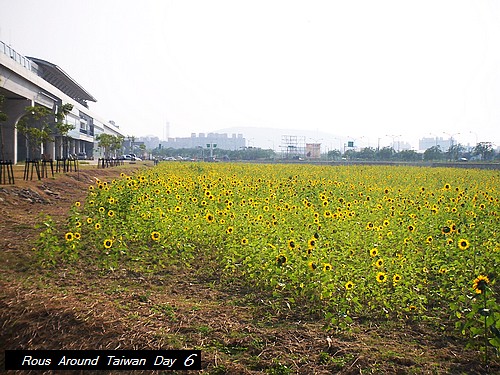This photograph, captioned "Rous Around Taiwan Day 6" in white text at the lower left corner, showcases a field of small sunflowers with green stalks and vibrant yellow petals around black centers. The field is surrounded by brown soil, and there are areas where the dirt is cleared, especially on the sides. The left-hand side of the image features some stools or planters around trees. In the background, a large building, likely a stadium or event center, is visible. There's a highway with cars and additional industrial buildings further in the distance. The scene is enveloped in a gray, misty, or smoggy atmosphere, with a hazy sky that filters the sunlight.